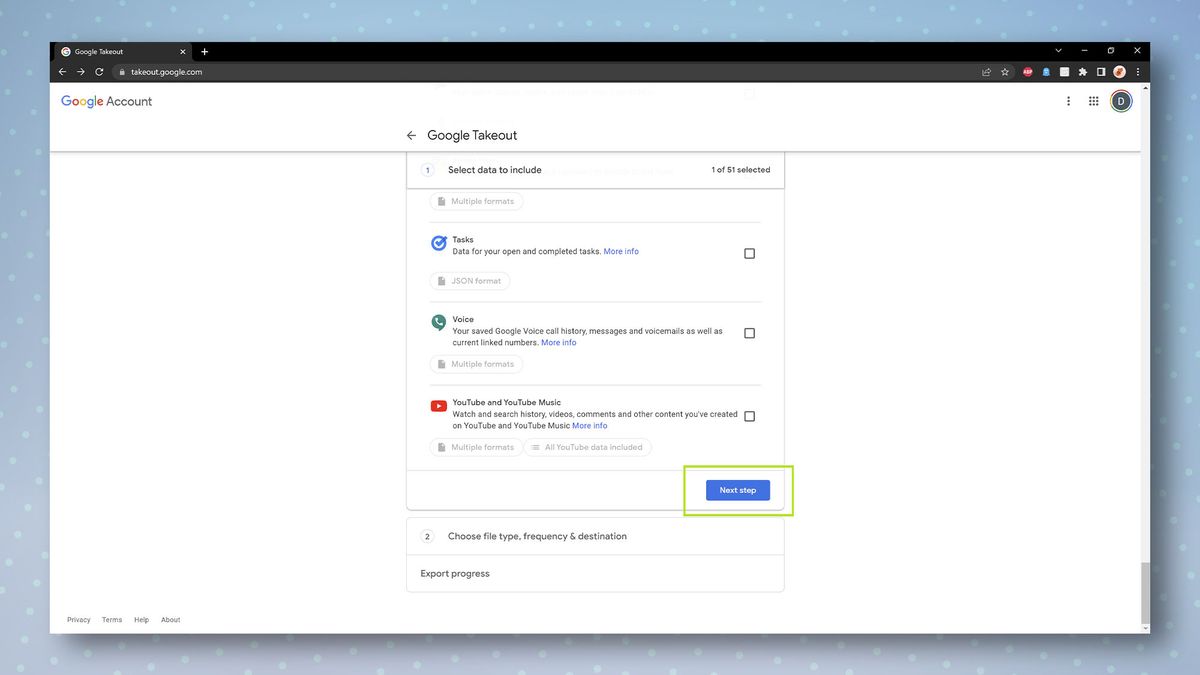The image depicts a predominantly white background of a webpage displayed on a computer screen. The content primarily consists of black text. At the top of the page, there is a banner featuring various navigation icons, including an 'X' for closing the window, a printer icon, among others. Below this banner is a secondary menu bar with several tabs and additional local navigation icons. The text on the page indicates that it is related to a Google Account, specifically referencing the Google Takeout application. The font size of the text on the page appears to be quite small, making it difficult to read the finer details.